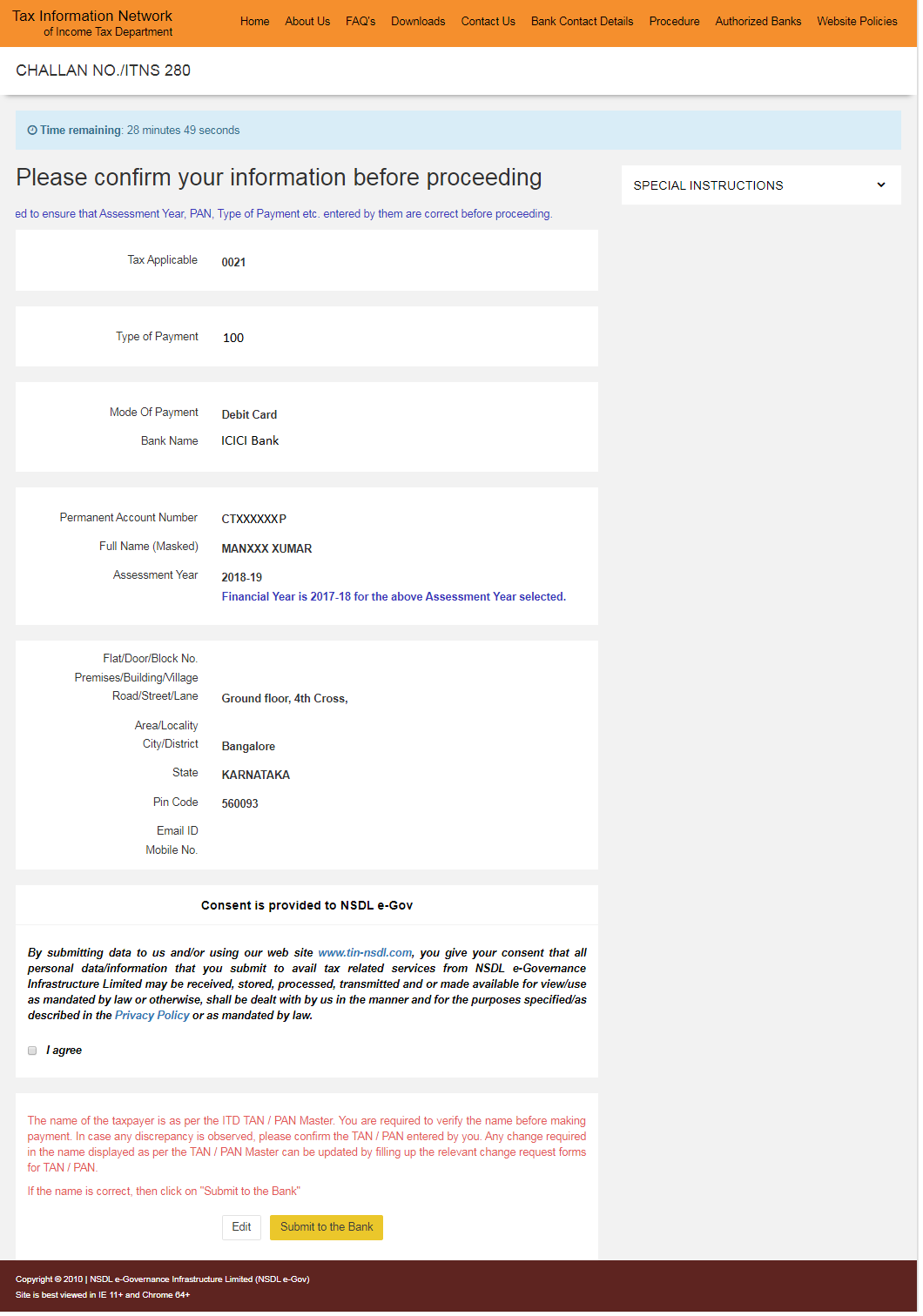The image features the Tax Information Network website. At the top, the header displays 'Tax Information Network' prominently. There is a series of navigation tabs including Home, About Us, FAQs, Downloads, and Contact Us. Additional tabs are Bank, Contact Details, Procedure, Authorized Breaks, Banks, and Website Policies.

Below the navigation tabs, essential sections are titled Challenge, NL/ITNS, and 280. A blue rectangle on the right side shows a countdown timer indicating 'Time Remaining: 28 minutes and 49 seconds'. 

The main content area prompts users with a message: "Please confirm your information before proceeding." Several input fields are available for users to fill in their details, such as:
- Tax Applicable
- Type of Payment
- Mode of Payment
- Bank Name
- Payment Account Number
- Full Name
- Assessment Year
- Email Address
- Home Address.

Each of these fields is likely accompanied by dedicated boxes where users can enter the required information to continue with their tax-related processes.